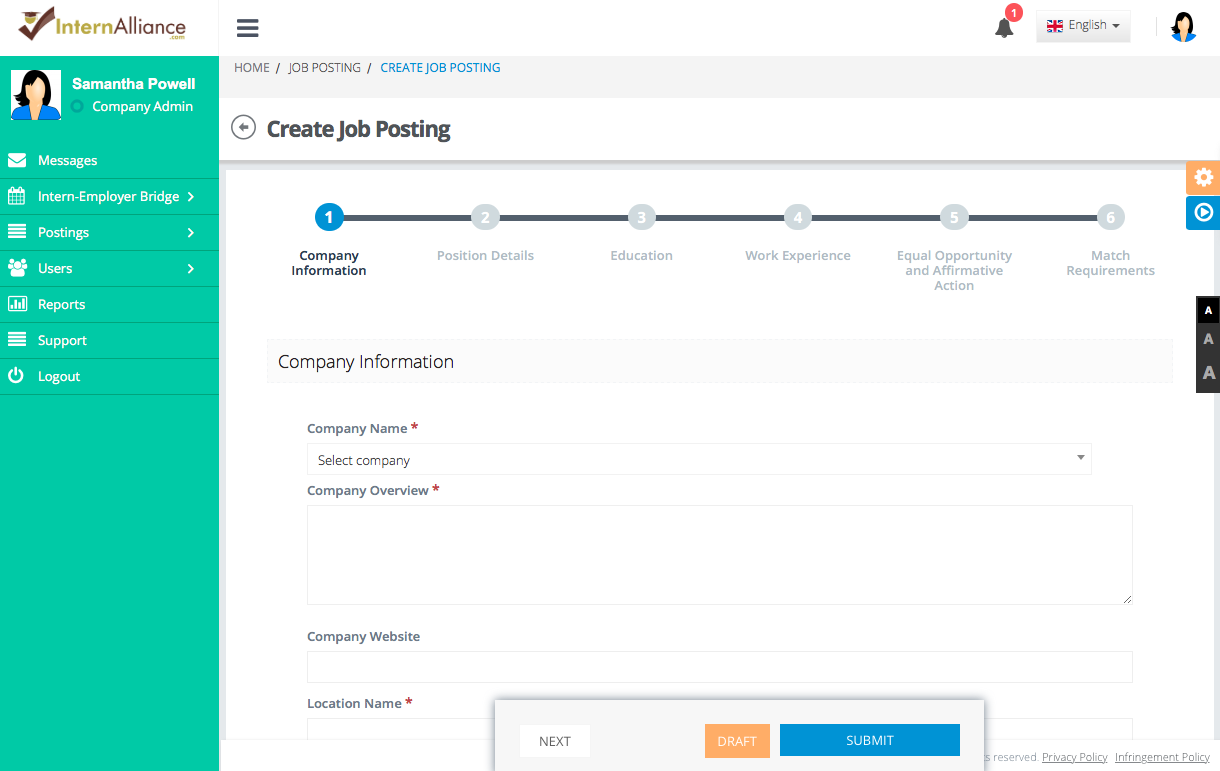On the top left of the page, the title "Intern Alliance" is prominently displayed. To the left, there is a sidebar featuring various options. At the top of this sidebar, it reads "Samantha Powell, Company Admin," accompanied by a generic, faceless cartoon image of a woman in a blue business-casual top. Below, a menu lists the following sections: Messages, Intern Employee Bridge, Postings, Users, Reports, Support, and Logout.

The main section of the page is organized into several subsections, beginning with Home, and followed by Job Postings and Create Job Posting. The user is currently on the "Create Job Posting" page, engaged in the process of creating a new job post. The form requires the user to enter various details segmented into six steps. The first step is "Company Information," which requests details like the company name, overview, website, and location. The subsequent steps are:

1. Company Information
2. Position Details
3. Education
4. Work Experience
5. Equal Opportunity and Affirmative Action
6. Match Requirements

At the bottom of the form are buttons to either submit or save the draft, as well as an X button to exit. On the right side of the page, a widget allows for adjusting the font size. In the top right corner, there is an option to change the language, currently set to English.